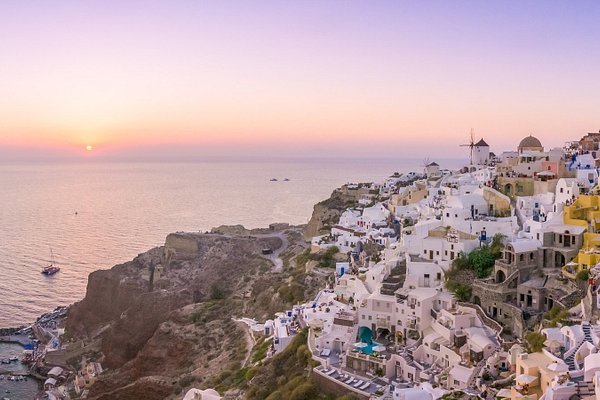This is a detailed photograph of a picturesque seaside town, likely in Greece, captured at sunset. The stunning scene features calm, blue water with a few small boats scattered in the distance, lending a serene backdrop to the vibrant coastal life. On the left side of the frame, the bright orange ball of the sun sets, casting a pink and lavender hue across the horizon and blending into the gradient of the sky, which transitions from light blue near the horizon to a rich lavender-purple at the top.

The main focus of the image is the hillside town situated along steep, rocky cliffs. These cliffs, brownish in color, are particularly steep at the bottom left where they meet the shore, adorned with some small white buildings. The town itself is densely packed with mostly white, cream, and gray buildings, interspersed with some deep yellow structures, creating a visually striking scene. The buildings appear quite old, with some likely serving as hotels, evidenced by the lounge chairs placed in front of them.

Adding to the picturesque architecture, there is a white cylindrical windmill with a brown, pointy roof and visible arms on the right-hand side of the image, atop the hillside. Nearby, a distinctive domed building marks the highest point of the town. The overall image showcases a beautiful blend of natural and architectural elements, enhanced by the rich, warm colors of the setting sun.